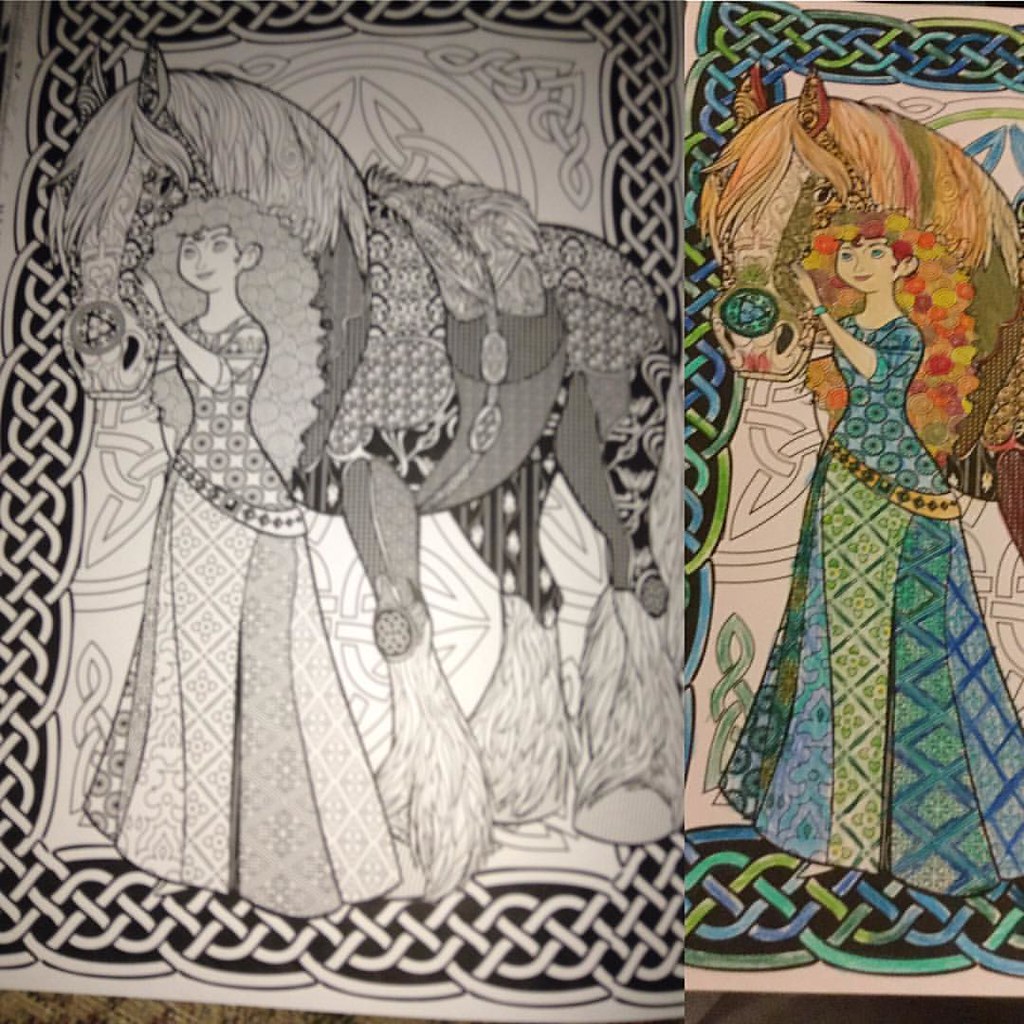The image consists of two side-by-side panels, each depicting the same intricate drawing sourced from a coloring book. The left panel presents the original, uncolored illustration of a regal princess standing beside her horse. Both the princess and her steed are adorned in elaborate attire, with a backdrop that includes a decorative banner featuring various emblems. Though slightly out of focus, the detailed linework of the drawing remains evident. In contrast, the right panel showcases the same image, now vividly colored. The princess's dress has been adorned with shades of gold, green, and blue, while her horse sports a striking green coat. The princess's hair is depicted as a flowing blonde, and the entire scene is framed by a border embellished in blue and green hues. This vibrant transformation highlights the ornate quality of the original illustration, bringing it to life with a rich palette.